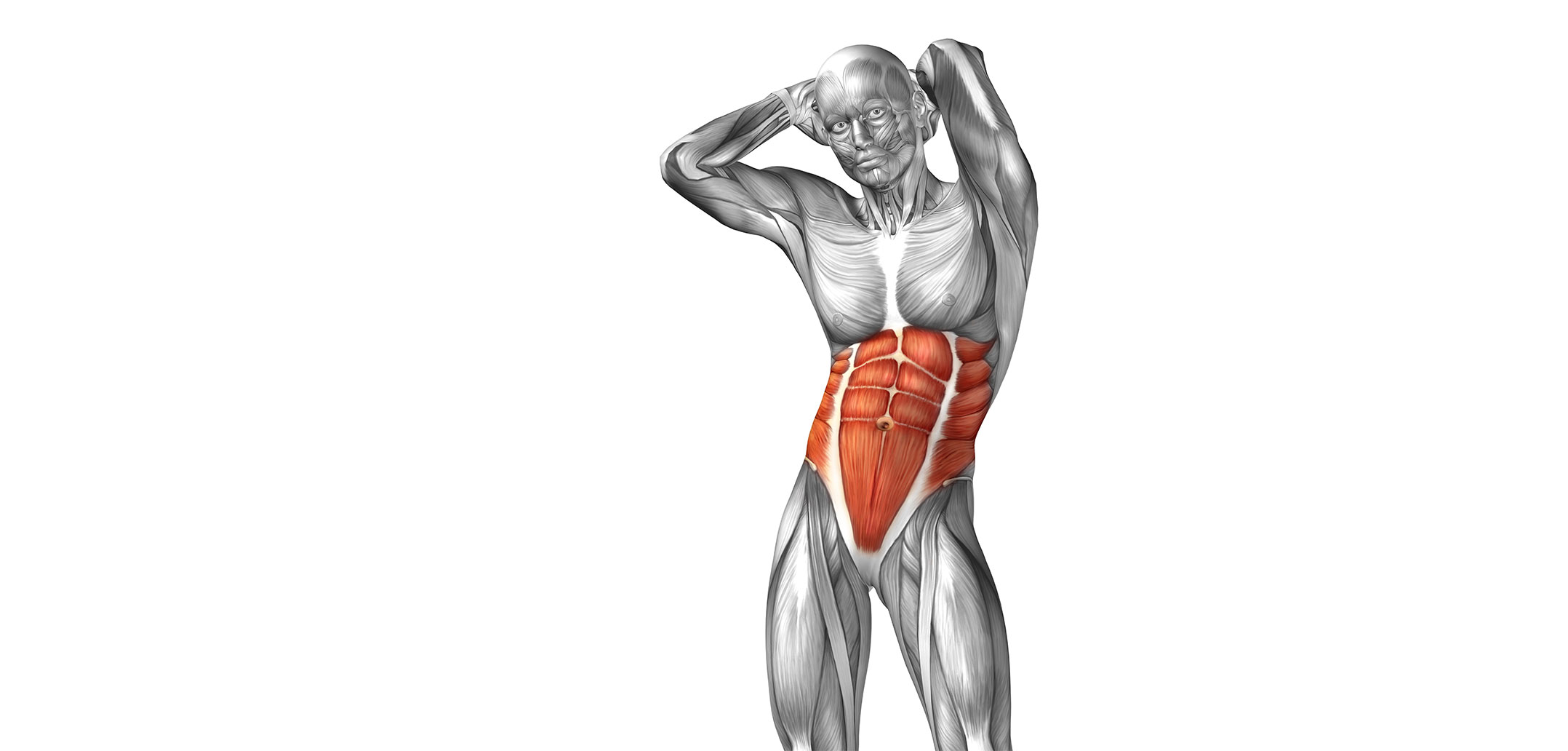This is a detailed anatomical illustration of a human figure depicted without skin, showcasing the intricate musculature of the body. The illustration is primarily rendered in shades of gray, silver, white, and black, with the notable exception of the abdominal region, which is highlighted in orange-red tones with a pink navel. The figure's head is bald and skinless, with visible eyes, and the facial expression is neutral. Both hands are raised and clasped behind the head, with elbows bent, giving a clear view of the muscle groups. The illustration captures the figure from the head down to just above the knees, meticulously emphasizing the core muscular regions, including a clearly defined six-pack and obliques in the abdominal area. The background is completely white, devoid of any additional elements or text, focusing solely on the anatomical details of the muscles. This type of pose is designed to illustrate the muscles engaged in such a position, with the coloration and detailing particularly accentuating the abdomen.